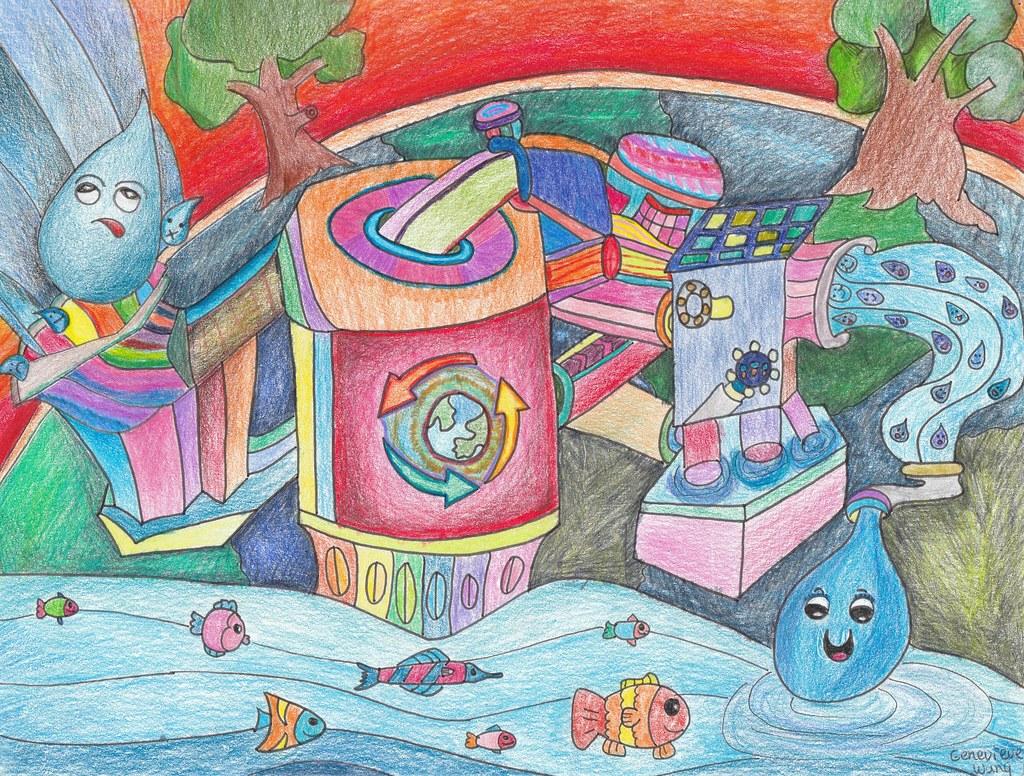The drawing appears to be a child's artwork, potentially created using colored pencils or watercolors. It vividly depicts an environmental scene where a river, colored blue, teems with multicolored fish of varying sizes. Alongside the river, there is an industrial complex that resembles a recycling or water processing factory, represented with a multitude of colors including red, pink, yellow, blue, and green. The factory features pipelines discharging water into the river, with some water droplets characterized by eyes and smiley faces. Additionally, a recycling logo, depicted as a globe with three arrows circling it in red, green, and yellow, is prominently displayed on the factory. The ground beneath the river and factory is curved, suggesting the shape of the earth, and adorned with trees that have brown trunks and green leaves. The overall scene, rendered in a cartoon-like, vibrant style, emphasizes environmental themes through its colorful and detailed composition.